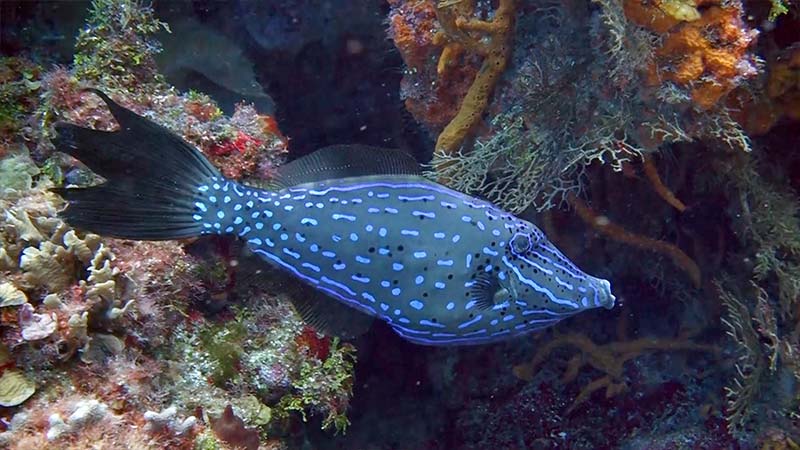This photograph captures a vivid underwater scene featuring a solitary tropical fish amidst a diverse coral reef. The fish, primarily a bright electric blue with dark green and silvery-grayish blue hues, showcases a striking elongated mouth that puckers, small eyes positioned on the sides of its face, and a long, three-pronged black tail. Its fins, blackish-green in color, add to its distinctive appearance. This colorful creature swims to the right against a backdrop teeming with various corals. The coral reef is jagged and vibrant, with clusters of orange, yellow, blue, gray, and even some pink and red corals and algae. Additionally, there are green plants sprouting and orange vine-like structures adorning the sea floor. The overall scene suggests either a natural underwater habitat or an aquarium exhibit, with the fish taking center stage in this brilliant aquatic tableau, sharply contrasted by the darker waters beyond the coral.